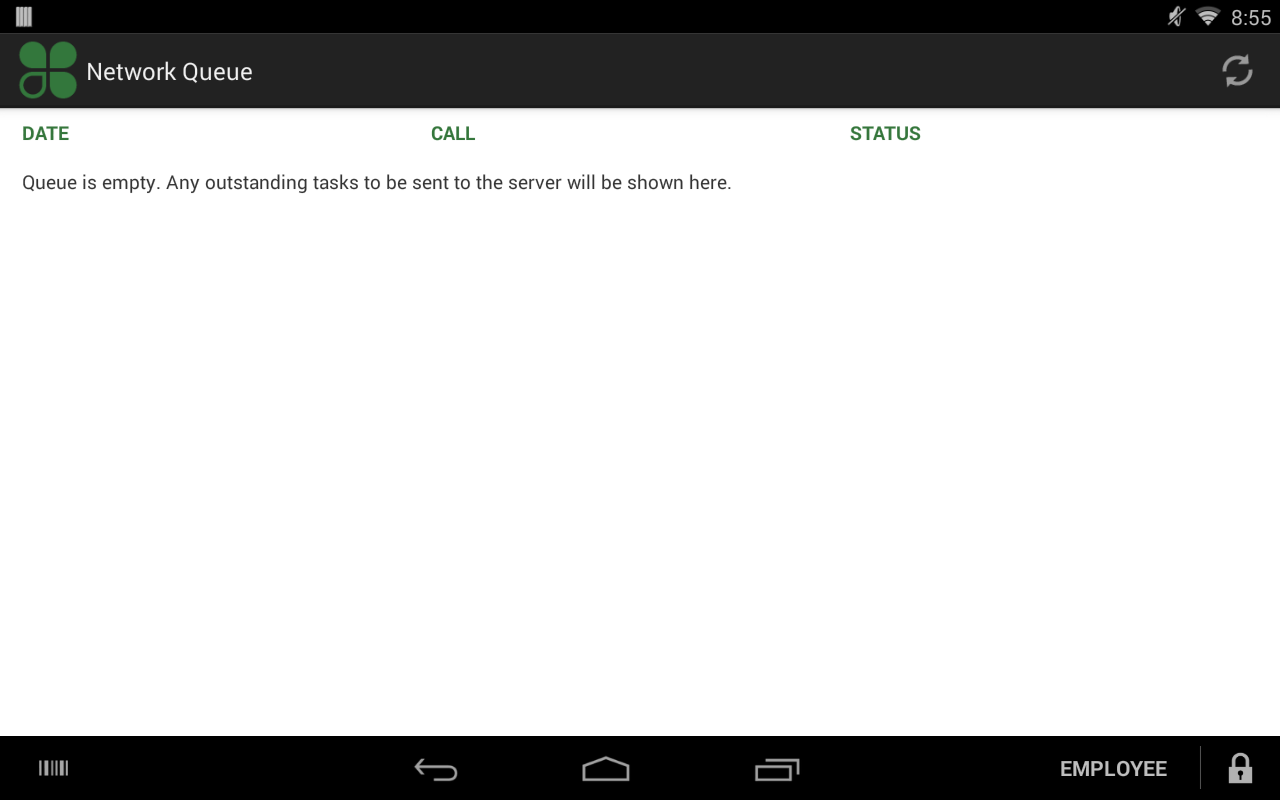In this image, a detailed screenshot of a tablet is displayed. The status bar, located at the top right corner, features several icons including a mute icon and a WiFi signal strength indicator showing 3 out of 4 bars. The current time on the device is 8:55. Below the status bar, there is a section labeled "network queue" which denotes that the queue is empty and any outstanding tasks to be sent to the server would appear here.

The tablet's interface also includes navigation keys at the bottom, with distinctly visible back, home, and recent apps buttons. The overall color scheme prominently features black and green. Additionally, there are references to an employee and a lock, indicating potential security or user-specific settings visible in the screenshot.